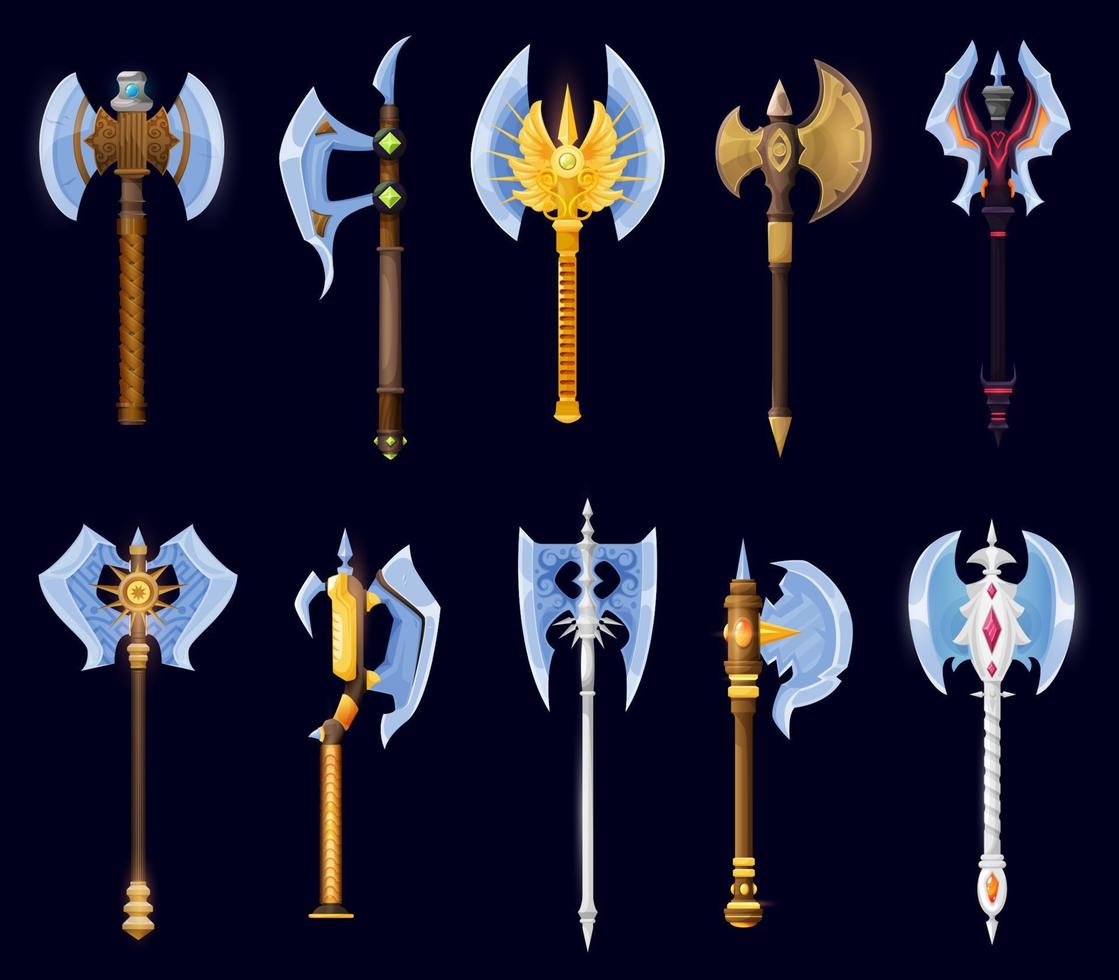This image depicts a detailed, cartoon-style illustration of ten ornate, fantasy-like axes arranged in two horizontal rows against a black background. Each row contains five axes. Most axes feature brown bases with a mix of gold and silver grips. The blades are predominantly light blue, resembling sharpened steel, though some unique pieces stand out—one with a gold and brown blade, positioned second from the right on the top row, and another with a bronze blade. The axes showcase varying designs: some have blades on both sides of the base, while others have a single, large blade on one side. Each axe is highly decorative, adorned with jewels, golden ornamentation, and spikes, giving them a formidable and weapon-like appearance. The top left axe is notable for its double-sided, round heads, reminiscent of a tomahawk. Despite their artistic and animated rendering, the detailed craftsmanship makes them look intimidating and battle-ready.